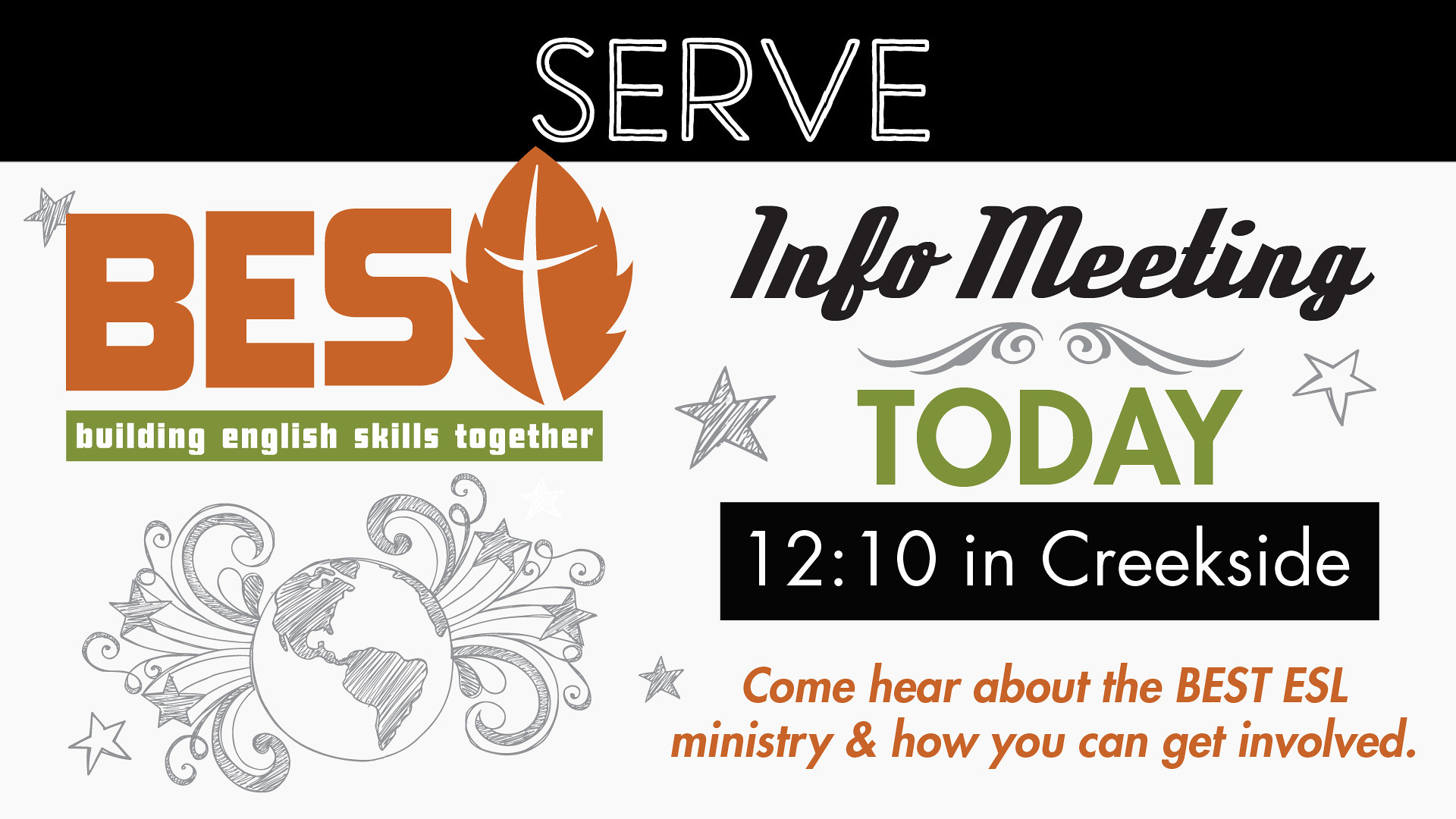The poster features a prominent black banner at the top with the word "SERVE" in all-caps white lettering. Directly below this is a white background with the letters "B-E-S" in bold orange, accompanied by an orange leaf with a white vein symbolizing the letter "T" in the acronym. Further down is a green banner with white text that reads "Building English Skills Together." Beneath this, there is a detailed sketch of the globe with stars and wavy patterns emanating from it. On the right-hand side of the poster, "Info Meeting" is displayed in black cursive, followed by "Today" in green text. Below that, a black banner with white print states "12:10 in Creekside." At the very bottom in orange text, the caption reads "Come hear about the BEST ESL Ministry and how you can get involved."